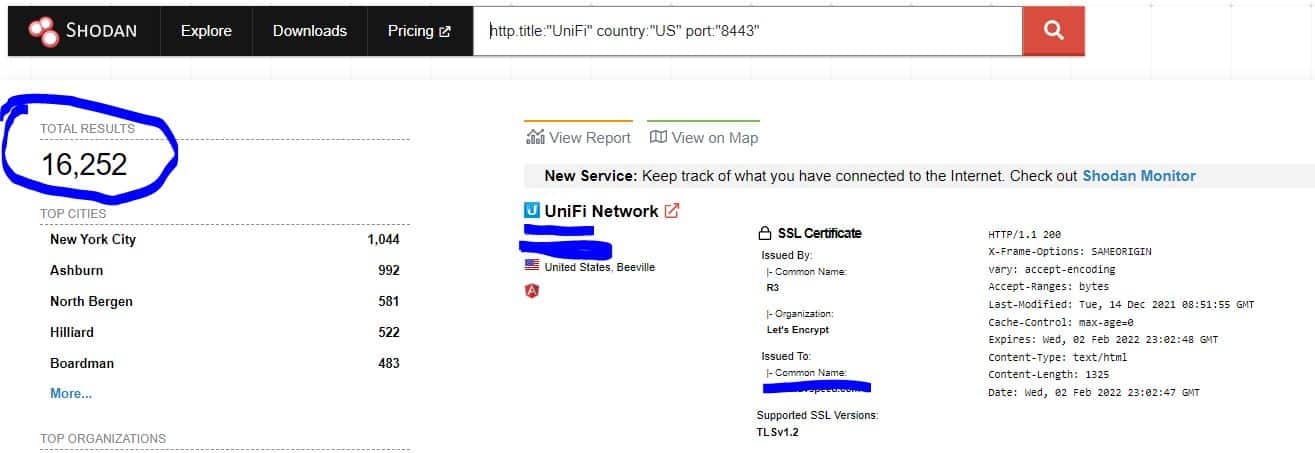A screenshot of the Shodan website's interface is displayed, showcasing various sections and functionalities. At the top of the page, a navigation menu includes options such as "Explore," "Downloads," and "Pricing." Below this, there is a search bar where a specific search query has been entered using advanced search operators. The query requires that the word "UNIFI" be present in the title, with results limited to the US and associated with port 8443. The search results indicate that 16,252 items match these criteria, which is highlighted with a red marker for emphasis. On the right side of the image, one of the search results is shown, titled "UNIFI Network SSL Certificates," providing detailed information related to technology and website security.